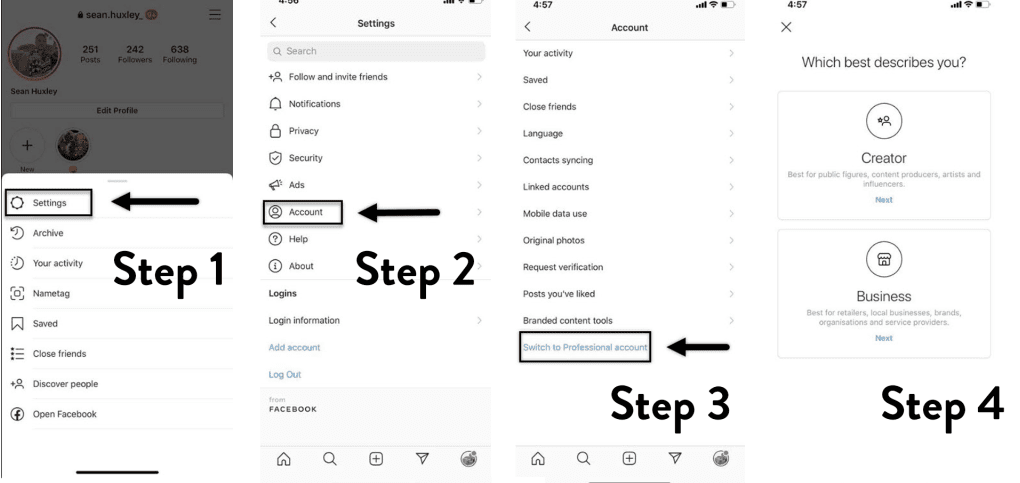Screenshot illustrating a four-step user interface with vertical boxes placed side-by-side on a white background:

**Box 1 (Step 1):**
- Displays a profile overview. 
- Top-left corner: Round profile picture of Sean Huxley.
- Center-top text: "Sean Huxley."
- Below the name: "251 posts, 242 followers, 638 following," and an "Edit Profile" option.
- Vertical menu options listed down the left side:
  - Settings
  - Archive
  - Your Activity
  - Name Tag
  - Saved
  - Close Friends
  - Discover People
  - Open Facebook
- A black horizontal line is present at the bottom.

**Box 2 (Step 2):**
- Focuses on the settings menu.
- Menu options listed:
  - Follow and Invite Friends
  - Notifications
  - Privacy
  - Security
  - Ads
  - Account (highlighted with a black outline and black arrow pointing left towards "Account")
- Additional options below the highlighted section:
  - Help
  - About
  - Logins
  - Login Information
  - Add Account
  - Log Out
  - Facebook.